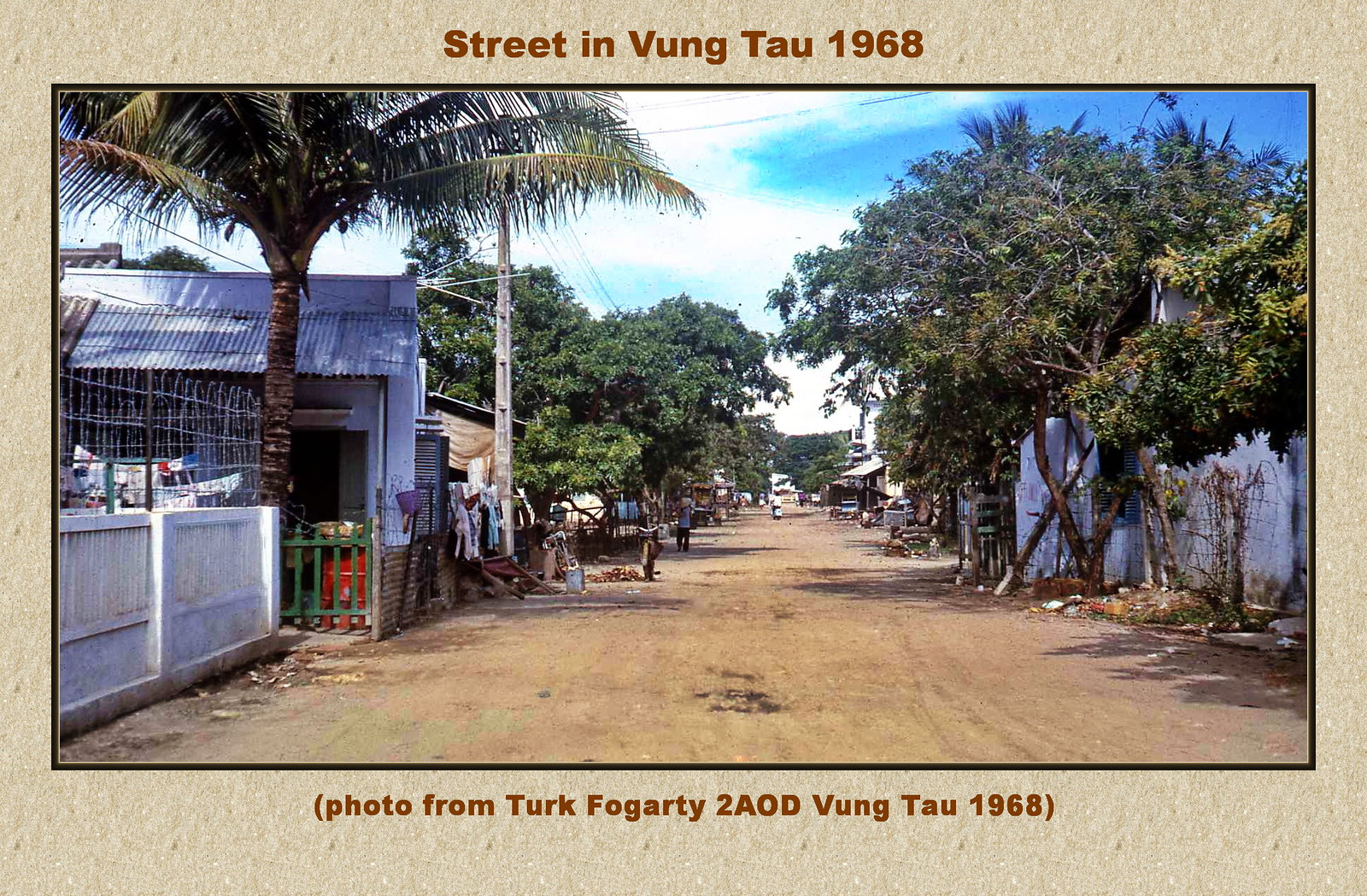This photographic image captures a vibrant yet seemingly impoverished street scene in Vung Tau, 1968. The photo is framed by a brown background with light brown text on top reading "Street in Vung Tau 1968" and similarly styled text at the bottom stating "(Photo from Turk Fogarty 2A OD Vung Tau 1968)." A solid black border surrounds the photo, enhancing its visual boundary. The setting is outdoors during the day, featuring a dirt road flanked by trees, including a prominent palm tree. On the right side of the street, there are fences, while the left side reveals more fences alongside a building with a corrugated metal roof. Additionally, a green fence and some wire mesh add to the makeshift aesthetic of the area. Clothes can be seen hanging out to dry, contributing to the lived-in feel of the scene. A telephone or power pole stands resiliently, and a couple of bicycles are parked on the left. Off in the distance, a man is riding a scooter alongside another man walking. The sky above is a beautiful blue with white clouds, adding a touch of serenity to the gritty surroundings. This detailed snapshot offers a glimpse into daily life in a modest community, marked by simplicity and resilience.